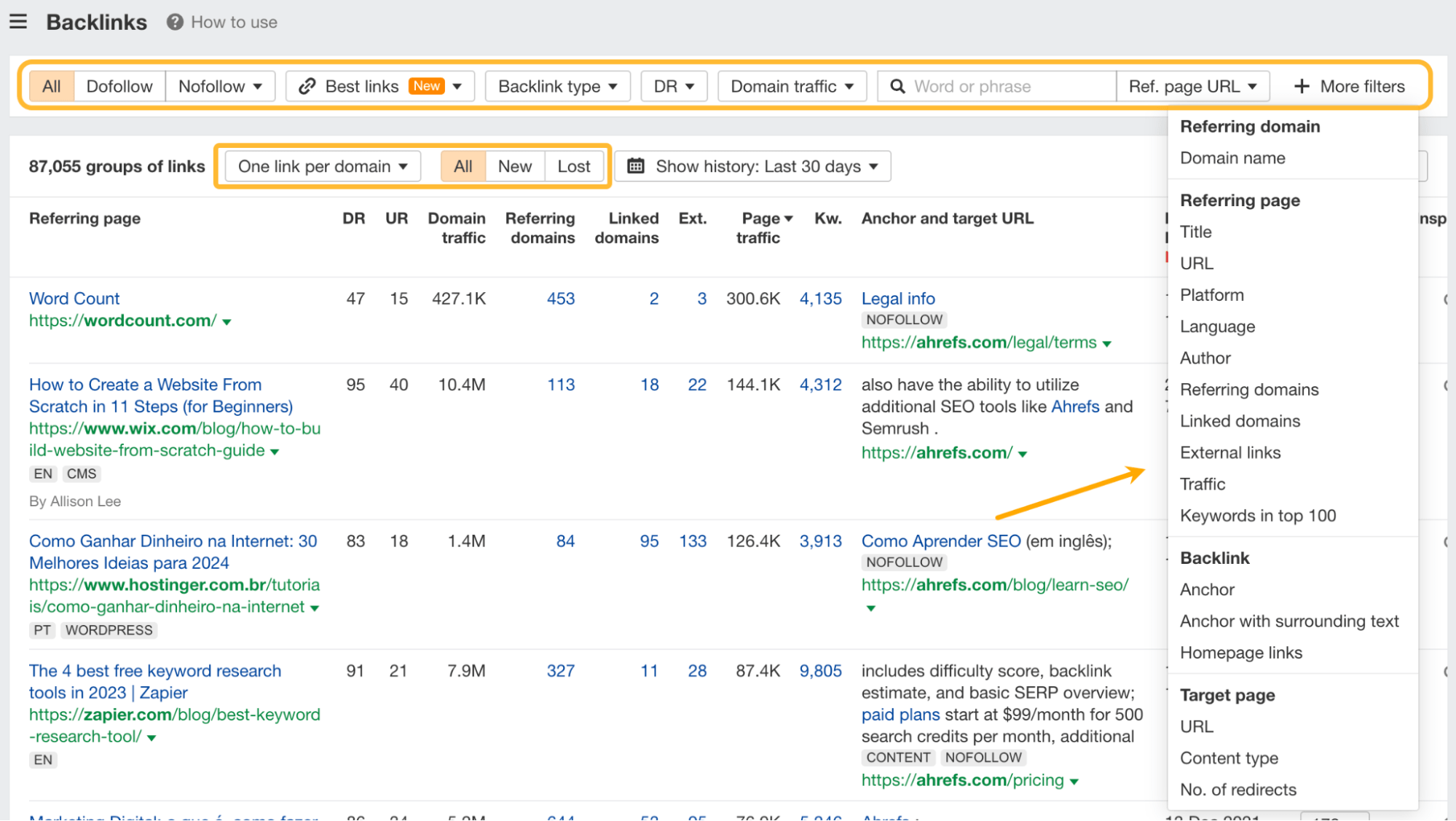This is a detailed and structured descriptive caption based on the provided voice input:

---

A computer screenshot displays a web page titled "Backlinks," with a small question mark icon next to the title indicating a help feature. The page has a gray background, and a prominent white overlay box is featured in the center of the screen. This overlay is divided into a narrow section at the top for dropdown selections and a larger section at the bottom, presumably for displaying results.

The top bar of the overlay box, highlighted with an orange outline, contains various dropdown options. It appears the user has expanded the "More filters" dropdown, which lists several filtering criteria vertically on the right side of the page, including "Traffic," "Keywords," "Title," and "URL."

On the left side of the overlay, there is a list of word counts and titles including:
1. "How to Create a Website from Scratch in 11 Steps for Beginners"
2. "Cómo ganar dinero de internet" (translated as "How to make money from the internet")
3. Another title in a different language, followed by 
4. "The Four Best Keyword Research".

An arrow originating from the title in a different language points towards the dropdown box, specifically highlighting the "External Links" option.